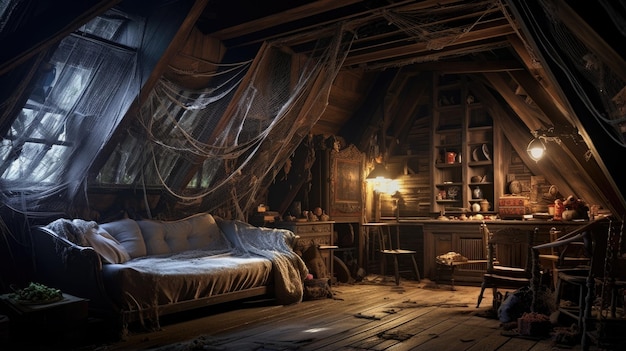The image depicts a realistic, computer-generated scene of a slightly eerie attic in an old wooden house. The attic features dark brown wooden floorboards and a v-shaped ceiling supported by large wooden beams, accentuating its rustic and aged appearance. On the left side of the room, beneath sloping windows framed in dark wood, sits a raggedy old couch draped with worn, white bed linens and cushions, all enshrouded in substantial cobwebs that stretch across the ceiling and windows. The right side of the attic is illuminated by bright yellow lantern lights, which highlight a cluttered scene that includes several wooden chairs and a desk area. A wooden cupboard with shelves, possibly storing red pots and gray plates, adds to the room’s antiquated charm, despite the mysterious and somewhat creepy atmosphere. The space also appears slightly chaotic, with clothes scattered on the floor, enhancing the unsettling, spooky vibe of this almost photographic illustration.